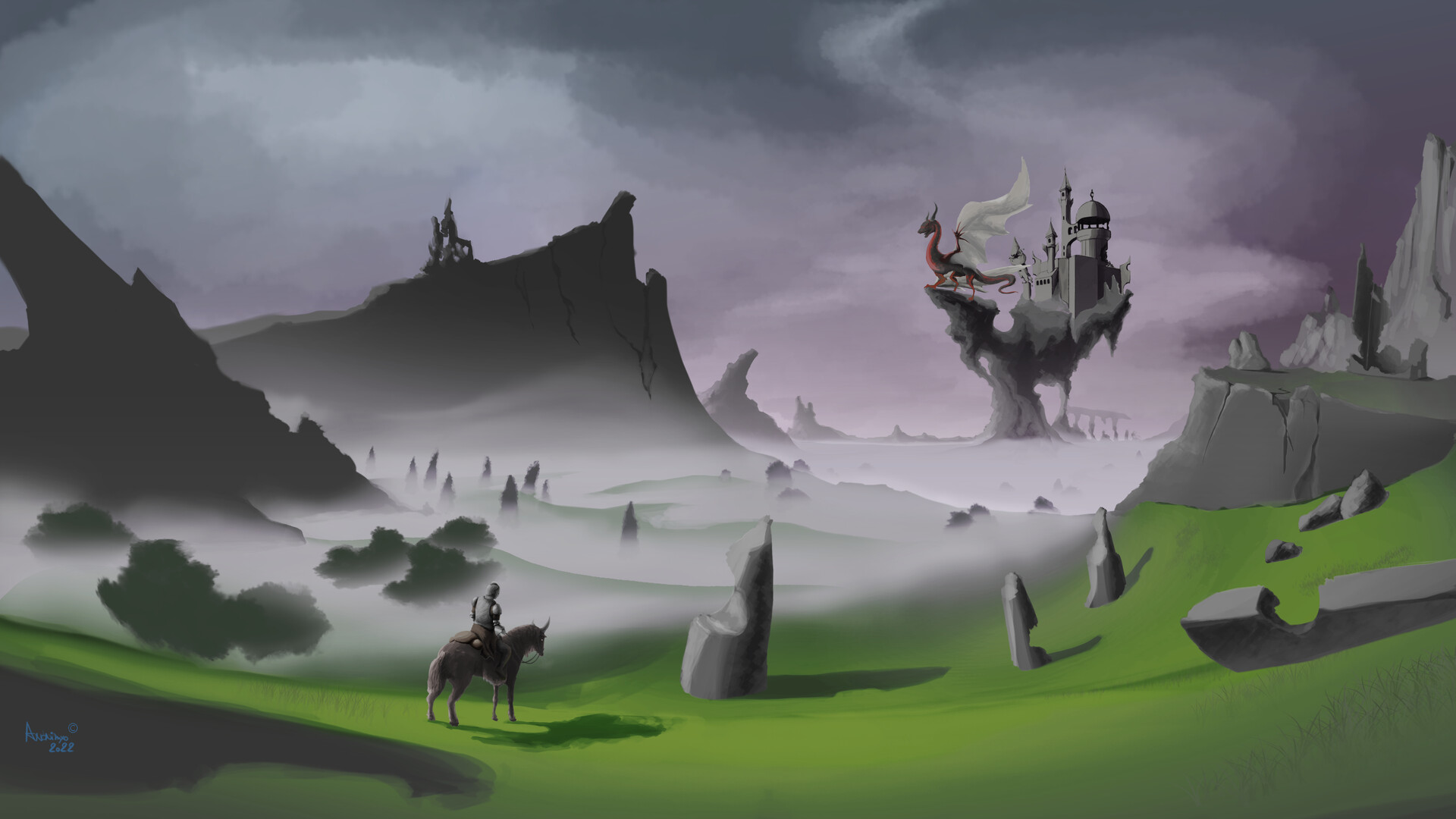The painting is a fantastical scene set against a mystical, swirling gray and purple sky. At the lower left center, a knight in a suit of gray armor sits astride a brown horse with a white tail, gazing intently into the distance. The horse stands on a patch of green grass, surrounded by scattered gray stones and bushes, with hints of fog weaving through the scene. The landscape features oddly shaped dark gray and black mountains and cliffs on either side, creating a surreal atmosphere.

In the middle of the background, there appears to be water with wavy white reflections and scattered dark gray rocks. A prominent mountain plateau rises in the distant background, topped by a majestic red and gray dragon with white wings. Beside the dragon stands a towering castle, characterized by a large rounded roof, several pointed towers, and a few windows, all depicted in shades of gray. The scene is further adorned with various stone structures and a small castle, accentuating the painting's intricate and imaginative nature.